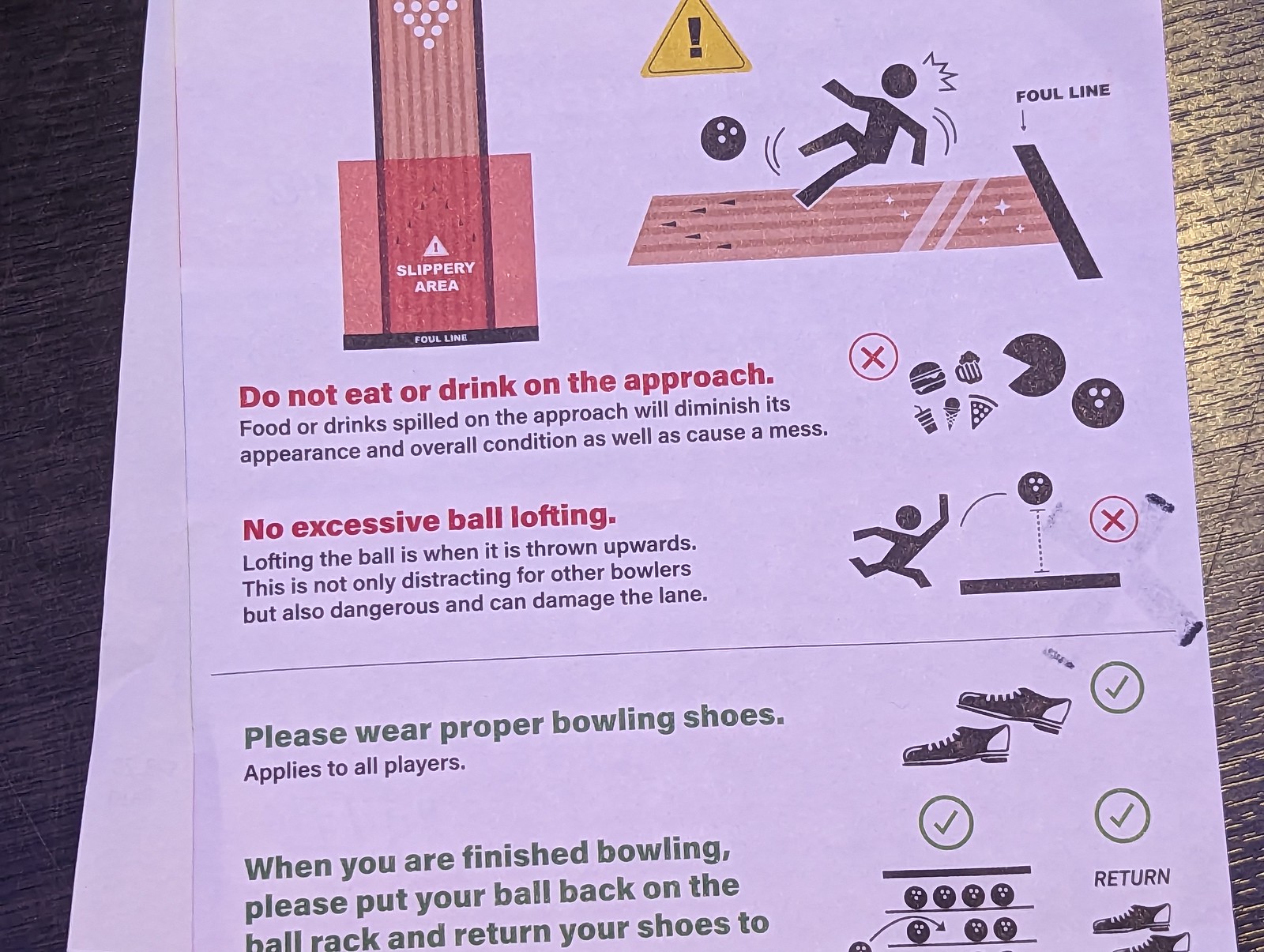The image showcases a detailed how-to manual and warning sign found at a bowling alley. This green-colored sign includes clear instructions and illustrations to ensure safety and proper etiquette while bowling. At the top of the sign is a diagram highlighting the slippery danger zone with a stick figure slipping near the foul line, emphasizing the importance of caution. 

Key rules are emphasized with bold, red text for the "no-no" behaviors and corresponding green check marks for proper conduct. The sign includes the following guidelines:
1. **Do Not Eat or Drink on the Approach**: Spilling food or drinks can damage the lane surface and cause hazards.
2. **No Excessive Ball Lofting**: Throwing the ball upwards can distract other players and damage the lane.
3. **Wear Proper Bowling Shoes**: Appropriate footwear is mandatory for all players.

Additionally, it reminds bowlers to return their balls to the ball rack and their shoes to the appropriate place when finished. The sign’s vertical layout features diagrams corresponding to each rule, providing visual reinforcement of the text instructions. The setting of this detailed informational sign is a bowling alley, depicted in a primarily beige, green, and red color palette with accents of black, white, gray, and orange.